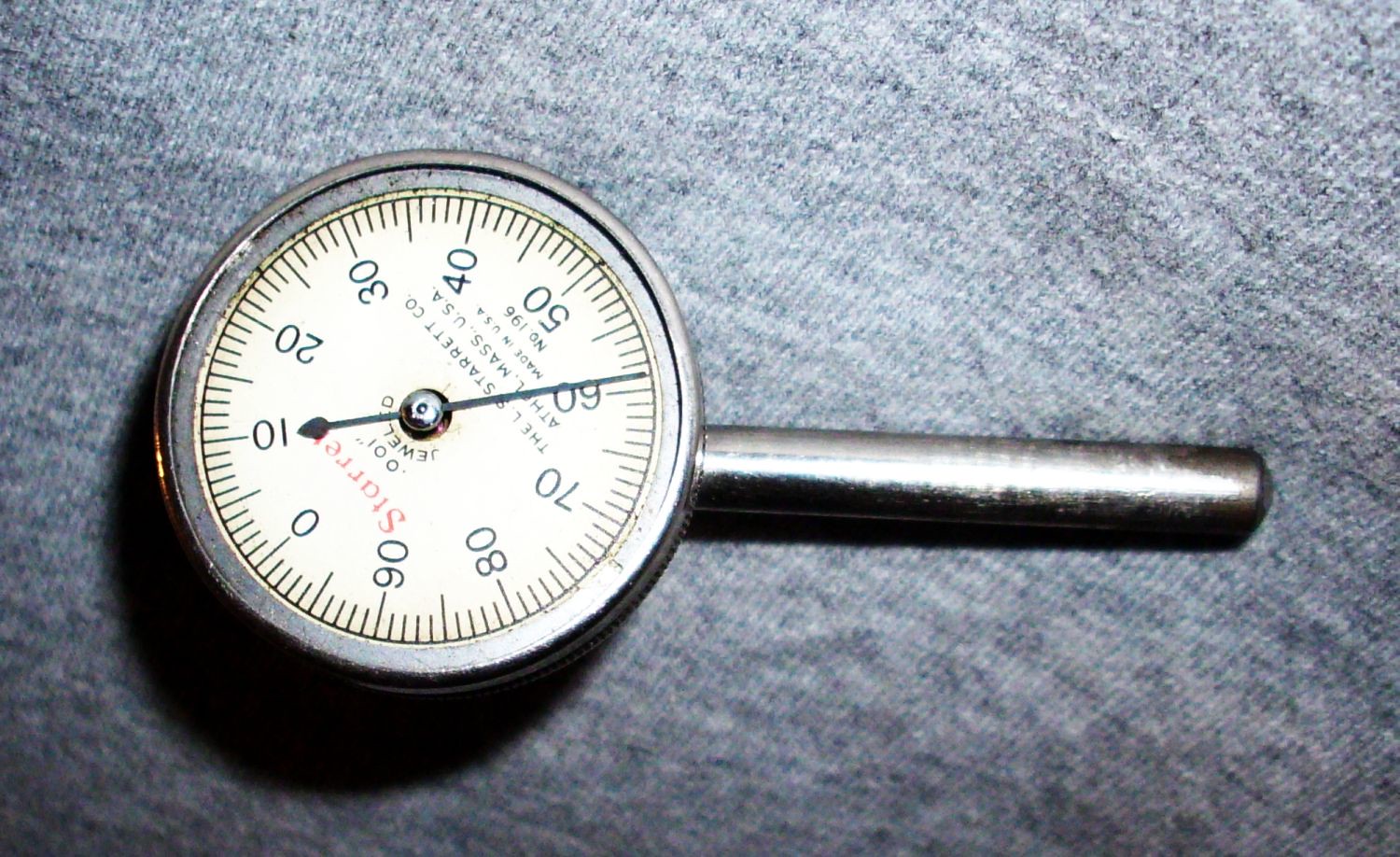Here's a cleaned-up and detailed caption for the image:

---

The image is a close-up of a metal pressure gauge placed on a piece of fabric with a denim-like texture. The fabric is predominantly gray, interspersed with flecks of green and other colors. The pressure gauge features a flat, cylindrical body made of metal, with a stem extending from one side. Its circular face is white, adorned with a series of numbers that increment in tens from 0 to 90 around its circumference. A needle on the dial is presently indicating the number 61. The meticulous composition and fine details suggest a focus on the precision and functionality of the device.